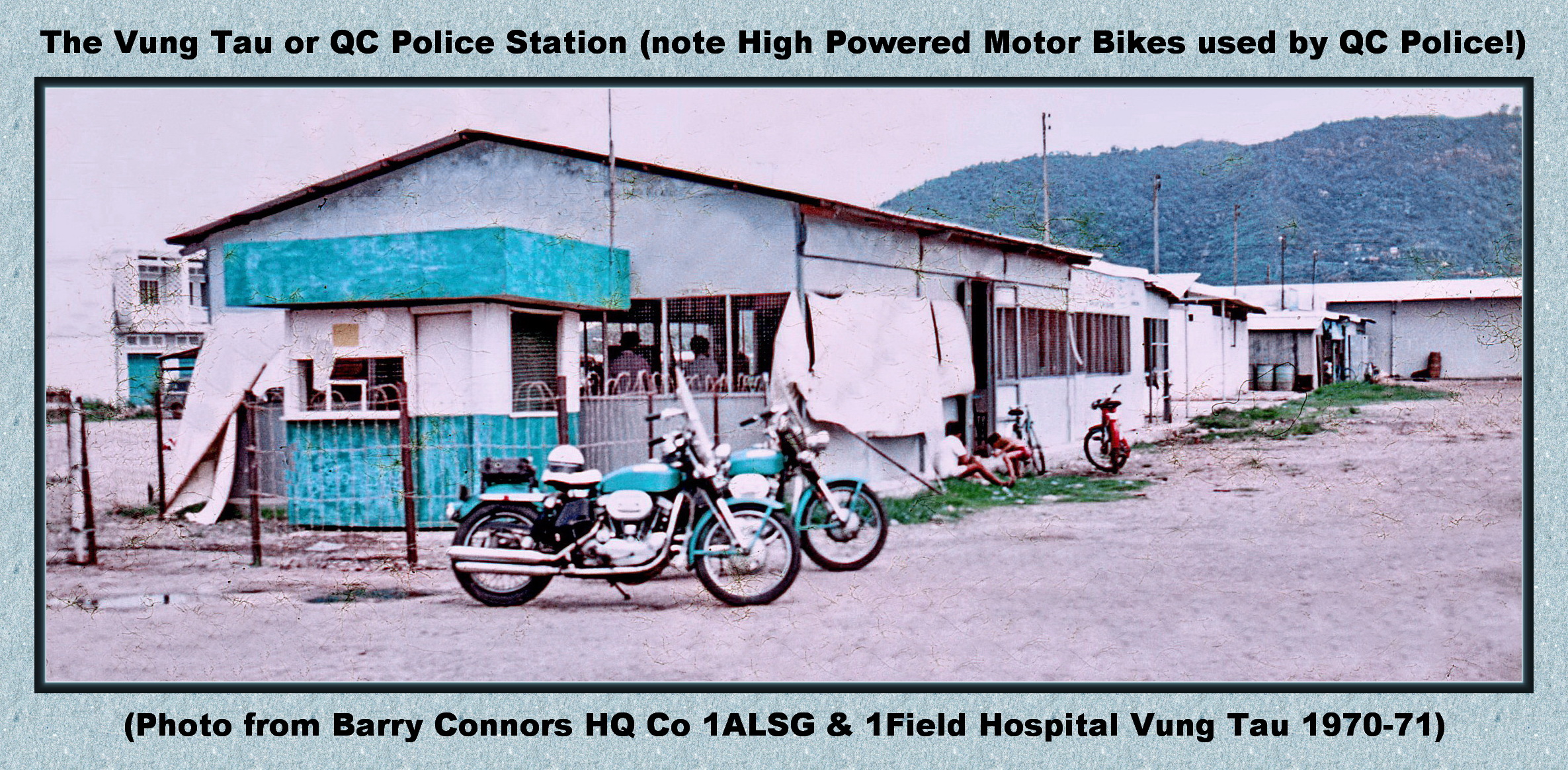The image depicts a vintage photograph centered within a light gray outline and framed by a black border. At the top of the image, black text reads, "The Vung Tau or QC Police Station (Note: High-powered motorbikes used by QC police)." At the bottom, it states, "Photo by Barry Connors HQ Co 1 ALSG and 1 Field Hospital Vung Tau 1970-71."

The photograph showcases a long, one-story police station with a white exterior marred by peeling paint revealing gray patches underneath. A teal-colored entrance is positioned on the left side of the building, featuring a door with matching teal and white sections and an open window beside it, providing a glimpse inside where people are visible.

In front of the station, there are two identical vintage motorcycles, one slightly offset to the left. Both bikes feature teal-colored gas tanks and fenders on the front and back tires, chrome exhausts, and windscreens. Further down the side of the building, a few smaller mopeds are parked on a patch of grass.

In the background, there is another white building, posts with power lines, and a mountain covered in green vegetation under a bright, clear sky. A few children are also visible on one of the building's steps, adding to the lively scene.